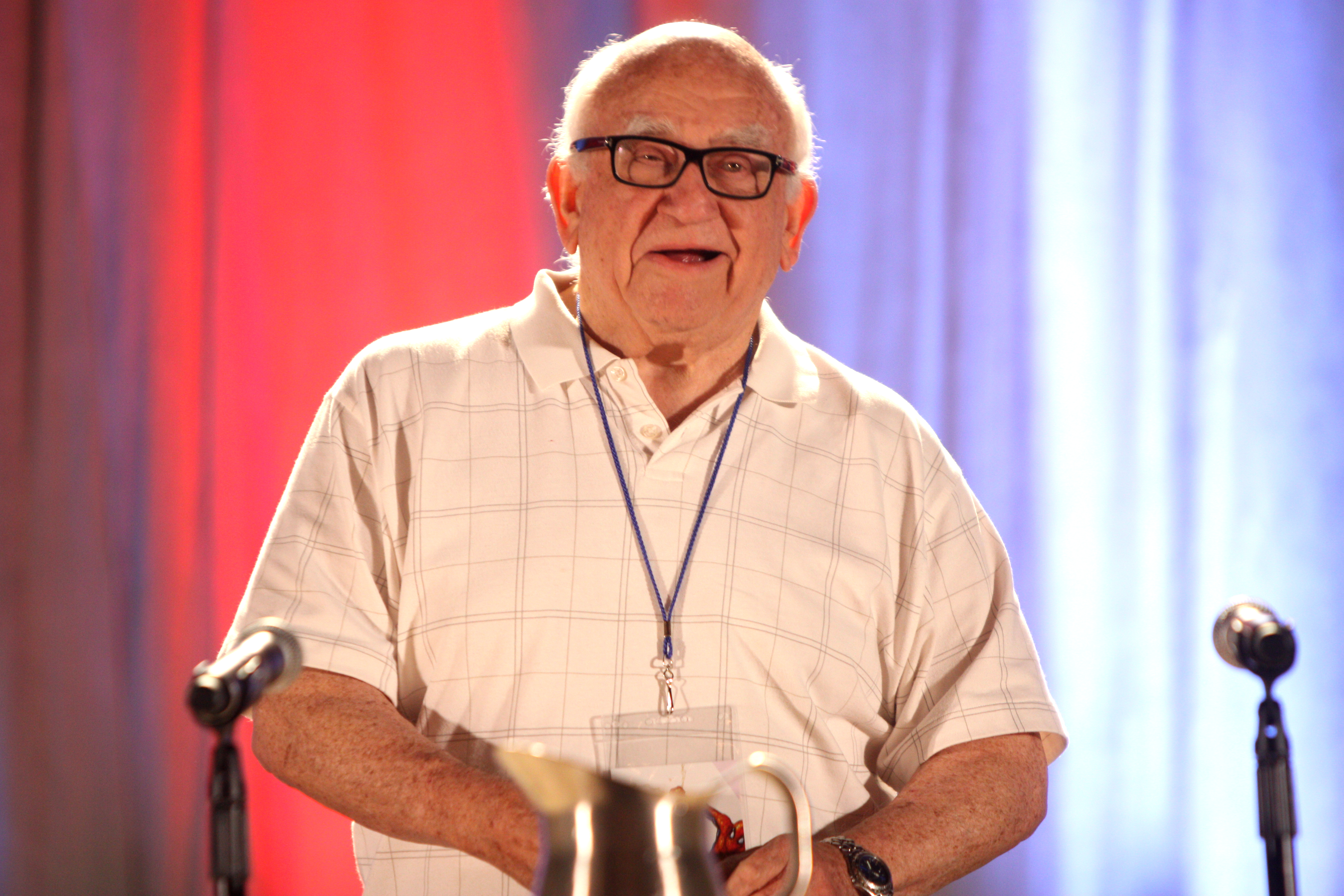The photograph features a man resembling Ed Asner, visible from his waist upwards with the rest of his body out of frame. He stands before a fabric curtain wall, divided into a pinkish-red section on the left and a whitish-blue section on the right. The man is dressed in a short-sleeved white shirt adorned with a black grid pattern, with the collar's two buttons undone. He wears a blue string lanyard around his neck, culminating in a clear plastic acrylic case containing a white card, which is concealed by his hands. His left wrist sports a watch, although this detail is somewhat obscured by a silver-colored pitcher situated nearby. 

Prominent in the image are two stand microphones, one in each bottom corner, both pointed towards the man. He is bald with gray hair flanking the sides of his head and sports thick-rimmed black glasses. His round face, adorned with spots and freckles similar to those on his arms, captures his expression mid-speech, with his mouth open as if talking.